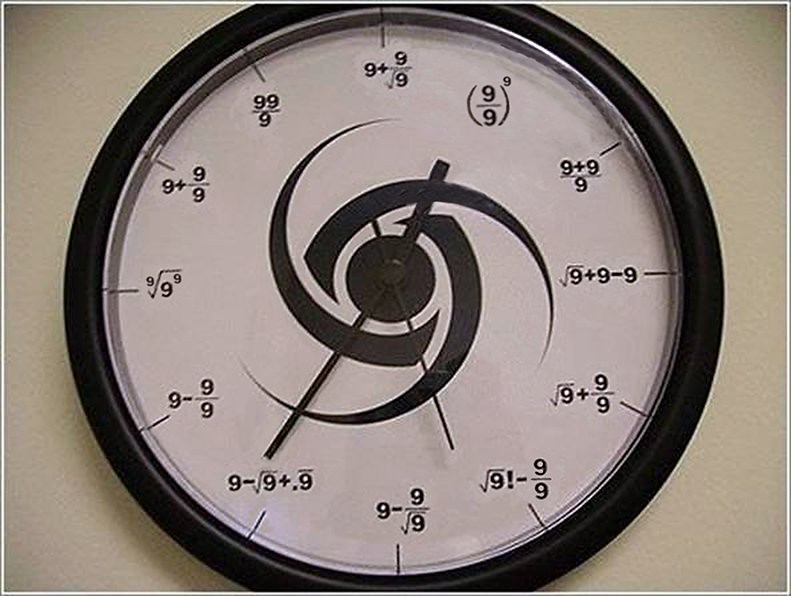This photograph showcases a unique novelty clock mounted on a pristine, white-painted wall, reminiscent of an office environment. The clock features a robust black trim encasing a transparent plastic cover, revealing an innovative design inside. Unlike traditional clocks, this one replaces standard hour numerals with mathematical equations, each resulting in the corresponding hour value.

The clock face is adorned with intricate equations involving addition, subtraction, division, and square roots, all with the theme of the number nine. For example, the position for the number one is represented by the equation "9 ÷ 9," while each hour mark follows a similar mathematical theme.

Currently, the hour hand points towards the position denoted by the equation for one, while the minute hand is positioned at the 35-minute mark. At the center of the clock face, a black circle anchors the hands, from which three stylized black extensions swirl outward, resembling talons or vortex patterns, adding an artistic touch to the clock's functionality.

This clock not only serves as a time-telling device but also as a mathematical curiosity and visual centerpiece, making it an intriguing addition to any wall.